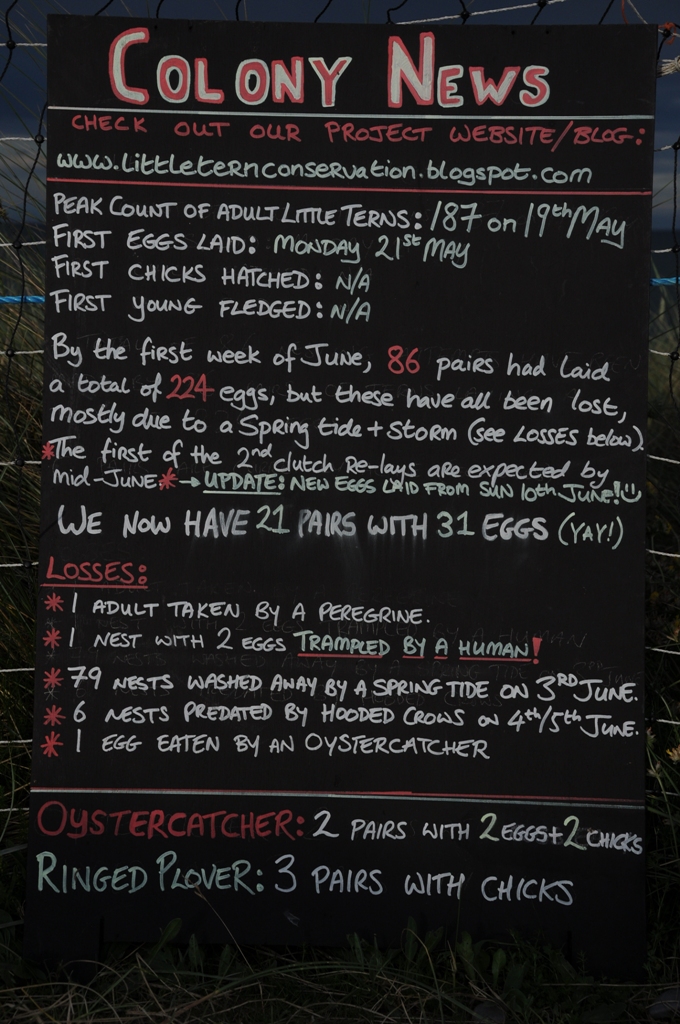The image depicts a weathered outdoor sign attached to metal rods, standing against a backdrop of tall grass on a cloudy day that hints at impending rain. The handmade sign, which appears to be personally crafted rather than computer-generated, prominently displays the title "Colony News." Beneath this, it invites viewers to visit the project website blog at www.littleternconservation.blogspot.com. Detailed updates include the peak count of adult little terns at 187 on 19th May, followed by the date of the first eggs laid on Monday, 21st May. The sign also notes initial milestones for first chicks hatched and first young fledged, which are marked as "N/A." It reports a significant loss of 224 eggs due to spring tides and storms by early June. However, it brings a hopeful update, mentioning new eggs laid by mid-June, specifically noting 21 pairs with 31 eggs as of Sunday, 10th June.